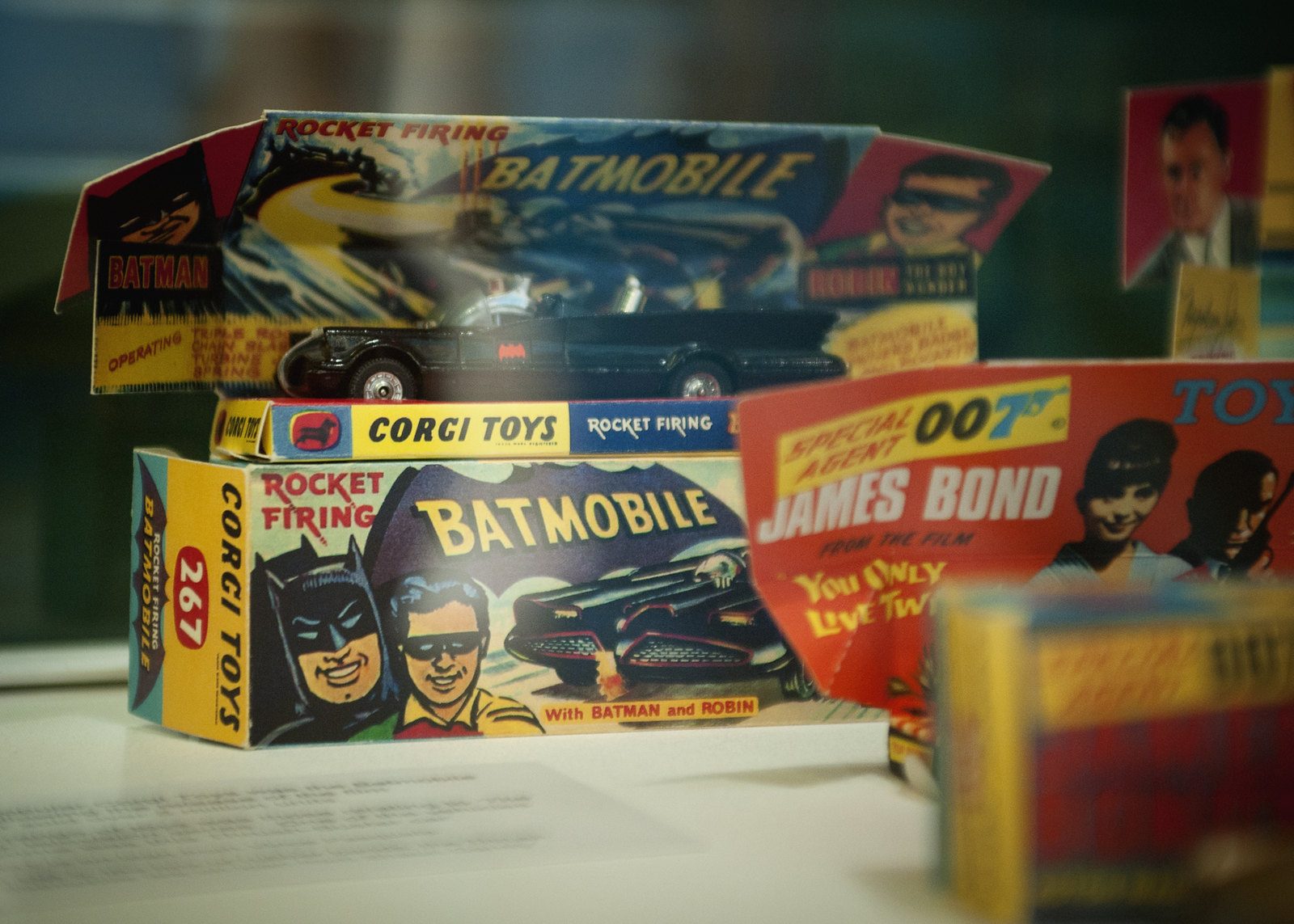This close-up photograph showcases a collection of vintage toy packaging set on a flat surface, partially obscured by a piece of paper with black writing. The focal point is a box for a Corgi Toys rocket-firing Batmobile, intricately designed in blue, red, and yellow. The Batmobile itself, accompanied by a small paper stand, sits atop the box. The packaging features vibrant images of Batman and Robin, with "rocket firing" prominently displayed. Additionally, the Batmobile box is labeled with "267" in a red circle. Flanking this is a red box labeled "Special Agent 007," featuring a blue gun-shaped '7' from the James Bond film "You Only Live Twice." This packaging includes an illustration of James Bond holding a gun alongside a woman in a blue dress. Another vintage toy package is present, but it remains out of focus and indistinct.